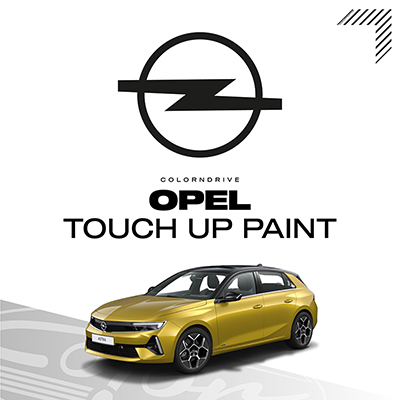The advertisement features a sleek gold-orange sedan with four seats, possibly a hatchback, prominently displayed against a clean white background. At the top, there's a distinct black logo, depicting a circle with a horizontally-oriented lightning bolt or "Z." Below the logo, the text "Color and Drive" is printed in black, followed by the term "Opel" in bold black font and then the phrase "Touch Up Paint" in regular black font. The car is angled toward the lower left corner, which is shaded gray and contains some indiscernible text. This section highlights a portion of the car painted in gray, drawing attention to the touch-up paint service being advertised.